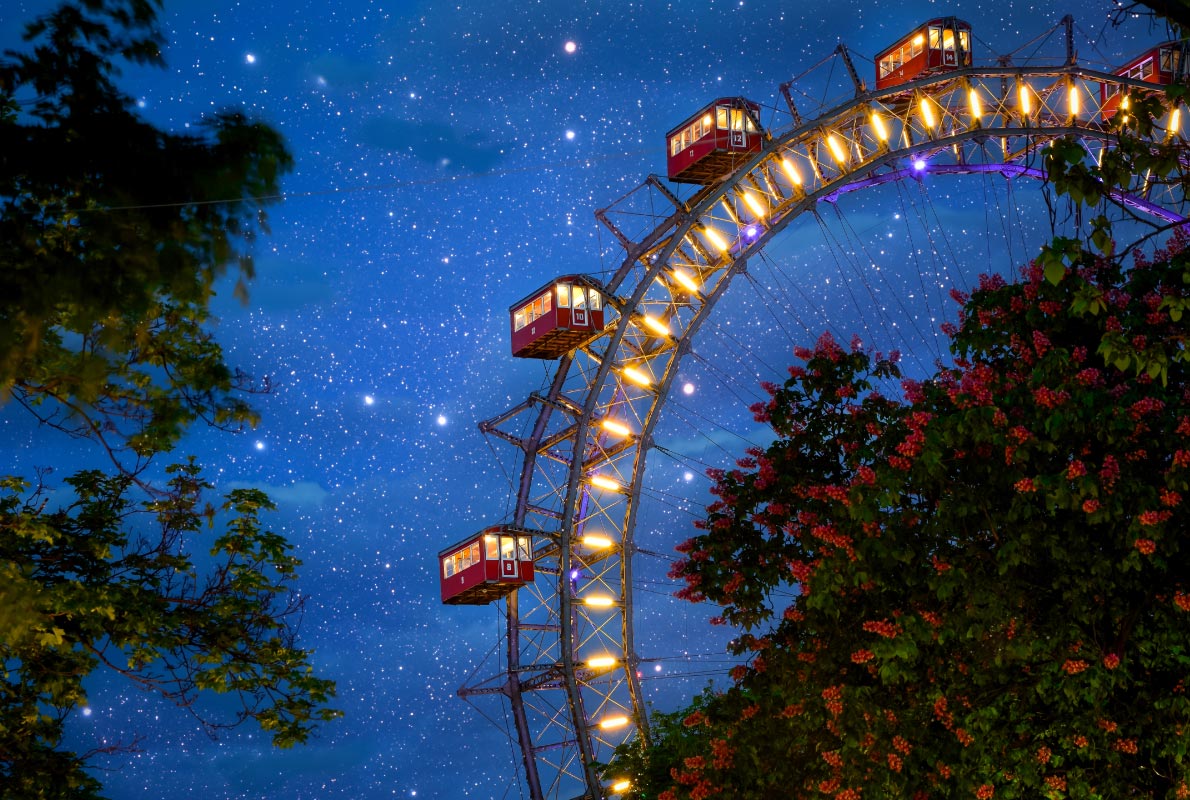This image captures a large Ferris wheel at night, set against a strikingly blue and star-studded sky. The Ferris wheel's carriages, which closely resemble trolley cars with windows all around and entry doors at the ends, are vividly red. These carriages are well-lit with purple and yellow lights, creating a vibrant display. In the foreground, to the right, there is a tree covered in clusters of red blossoms, while a standard green tree stands to the left. The combination of the illuminated Ferris wheel, the bright stars, and the colorful trees suggests this might be a scene from a festive carnival or a popular tourist spot.